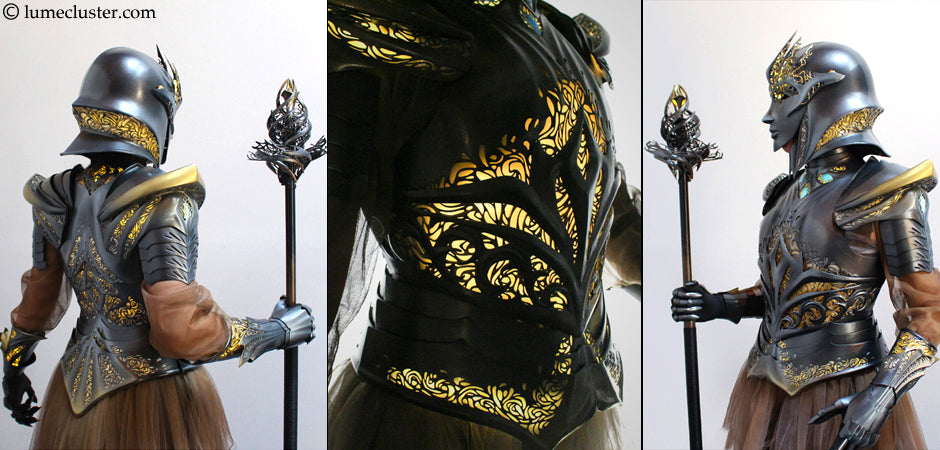This composite image features three detailed panels of intricately designed fantasy armor, presented side-by-side with black borders. In the upper left-hand corner, a black text watermark reading "copyright lumecluster.com" is visible. The left and right panels depict a woman clad in medieval-futuristic armor, showcasing both the front and back views of her torso. She wears a stainless steel helmet adorned with golden filigree and intricate woven patterns. Her upper body and shoulders are encased in similarly ornate armor, displaying a glowing yellow pattern that resembles roses. She is dressed in a loose, brown fabric dress with silver metal gauntlets on her hands, and completed with a decorative brown tulle skirt. Both images reveal her holding a distinctive staff with a dark black shaft, a copper handle, and an elaborate silver twist top that comes to a point. The central panel offers a close-up of the armor's breastplate under a darkened filter, illuminating the intricate golden filigree and glowing yellow detailing.